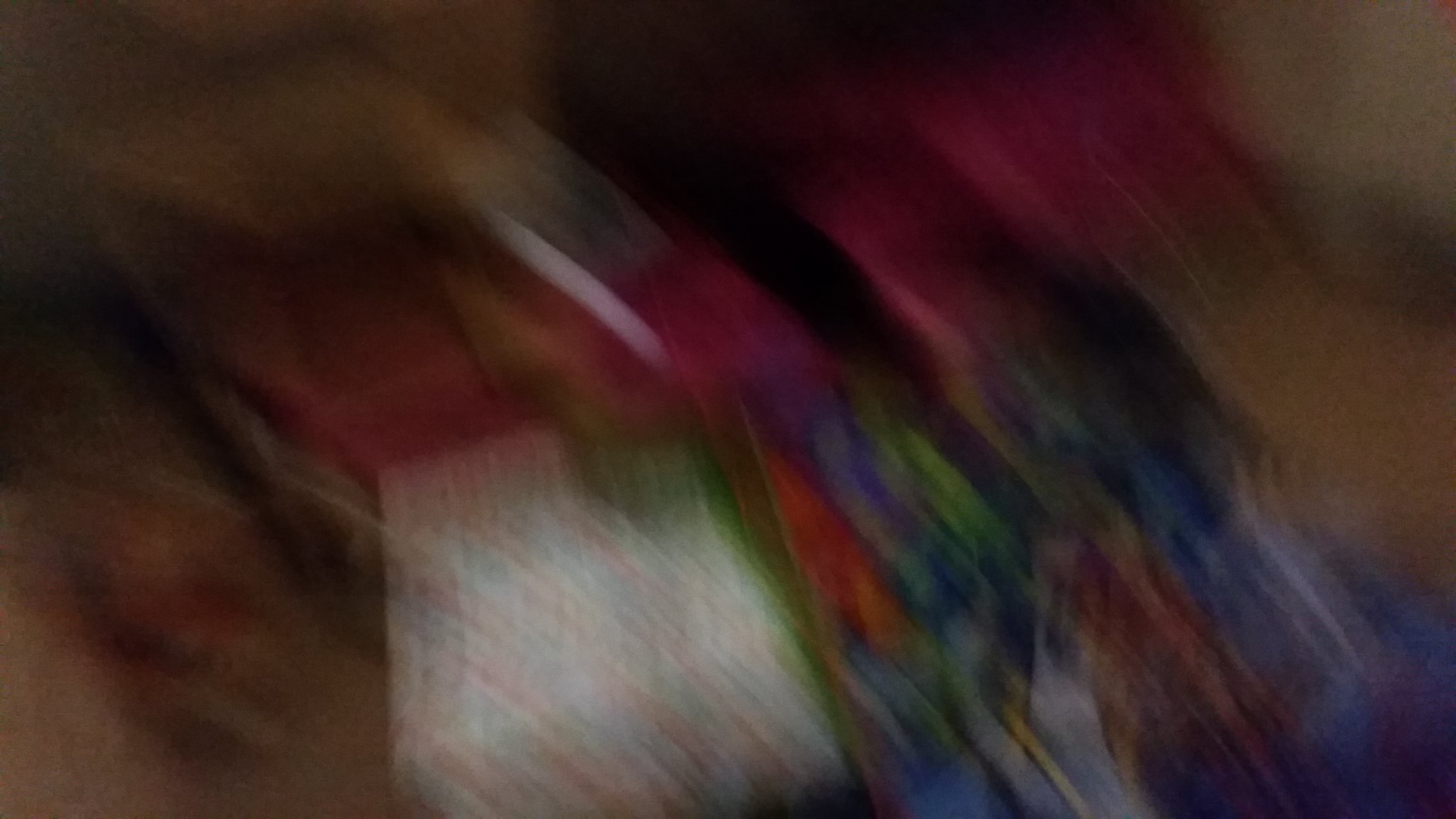This extremely blurry photograph appears to capture an abstract scene predominantly featuring various patches and streaks of vibrant colors. Near the lower left center, a white box is discernible, suggesting a downward viewing angle. The image is interspersed with several horizontal and diagonal lines in red and green, adding to the chaotic yet intriguing composition.

In the top left corner, a patch of magenta is bordered by a hazy brown hue, making that section particularly noticeable. Adjacent to the magenta on the right is a lighter segment of orange-yellow, seamlessly blending into another streak of magenta intersected by white. Continuing further right, additional patches of magenta merge with black, creating contrasting bands that enhance the image's dynamic feel.

The upper right corner displays a soft tan color, providing a subtle background to this vibrant mix. Finally, at the lower right of the white box, there are vertically angled patches of various colors such as red, orange, green, blue, gray, and white, adding a final element of complexity to this enigmatic, color-dappled composition.